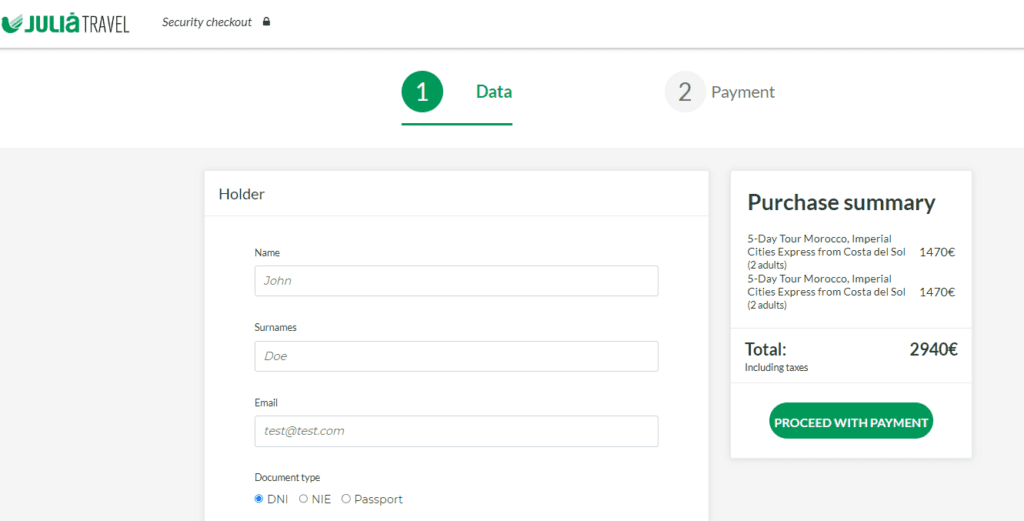A cropped screenshot from the Julia Travel website, featuring a form titled 'Holder' with blank fields for name, surname, email, and document type (options include DNI, NIE, or passport). Accompanying this form is a white box on the right, summarizing the purchase details: a five-day tour in Morocco for two adults, with a total cost of €2,940, including taxes. Above the form, the Julia Travel logo is displayed, with 'Julia' in green text and 'Travel' in black, beside a security icon indicating the website is securely encrypted. A green hyperlink is present to proceed with payment.